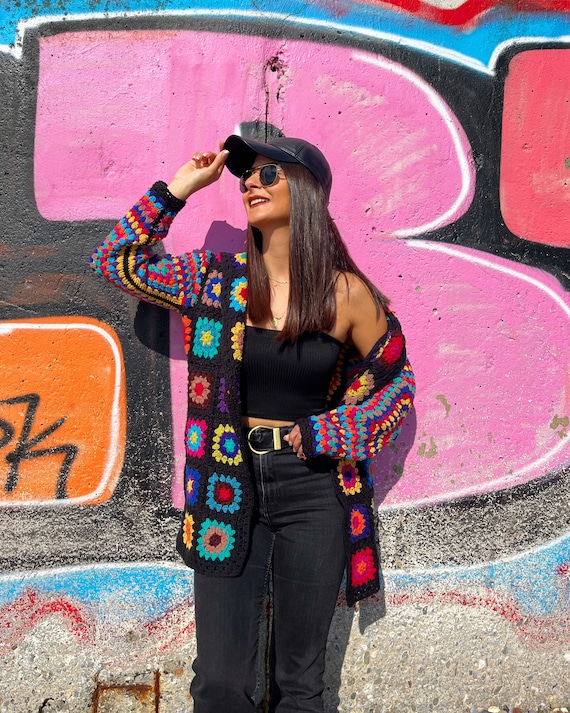This vibrant photograph features a smiling young woman posing confidently against a colorful graffitied wall. The wall itself is adorned with an array of bubbly and stylized graffiti in shades of pink, red, orange, blue, black, and turquoise, creating a vivid and dynamic backdrop.

The woman is an interesting focal point with her stylish ensemble. She has long, shiny, straight brown hair cascading down past her shoulders and is adorned with a black baseball cap, which she tips towards the sun with her right hand. Her fingernails are painted white, adding a touch of contrast to her look. She wears aviator sunglasses that hide her eyes but not her bright smile, accented by dark mauve lipstick.

Her outfit is carefully coordinated, featuring a black halter tube top that exposes her shoulders and midriff, and a pair of black skinny jeans held up by a thick black belt accented with gold detail. Adding a pop of color to her attire is a handmade crocheted cardigan with vibrant, patchwork-like floral and diamond patterns in hues of blue, purple, red, yellow, tan, and aqua. One side of the cardigan casually drapes off her arm, enhancing her laid-back, yet chic demeanor.

The photograph captures her in a relaxed pose, with her head slightly tilted and face uplifted to the sun, exuding a sense of joy and freedom as she stands against the backdrop of colorful graffiti art.